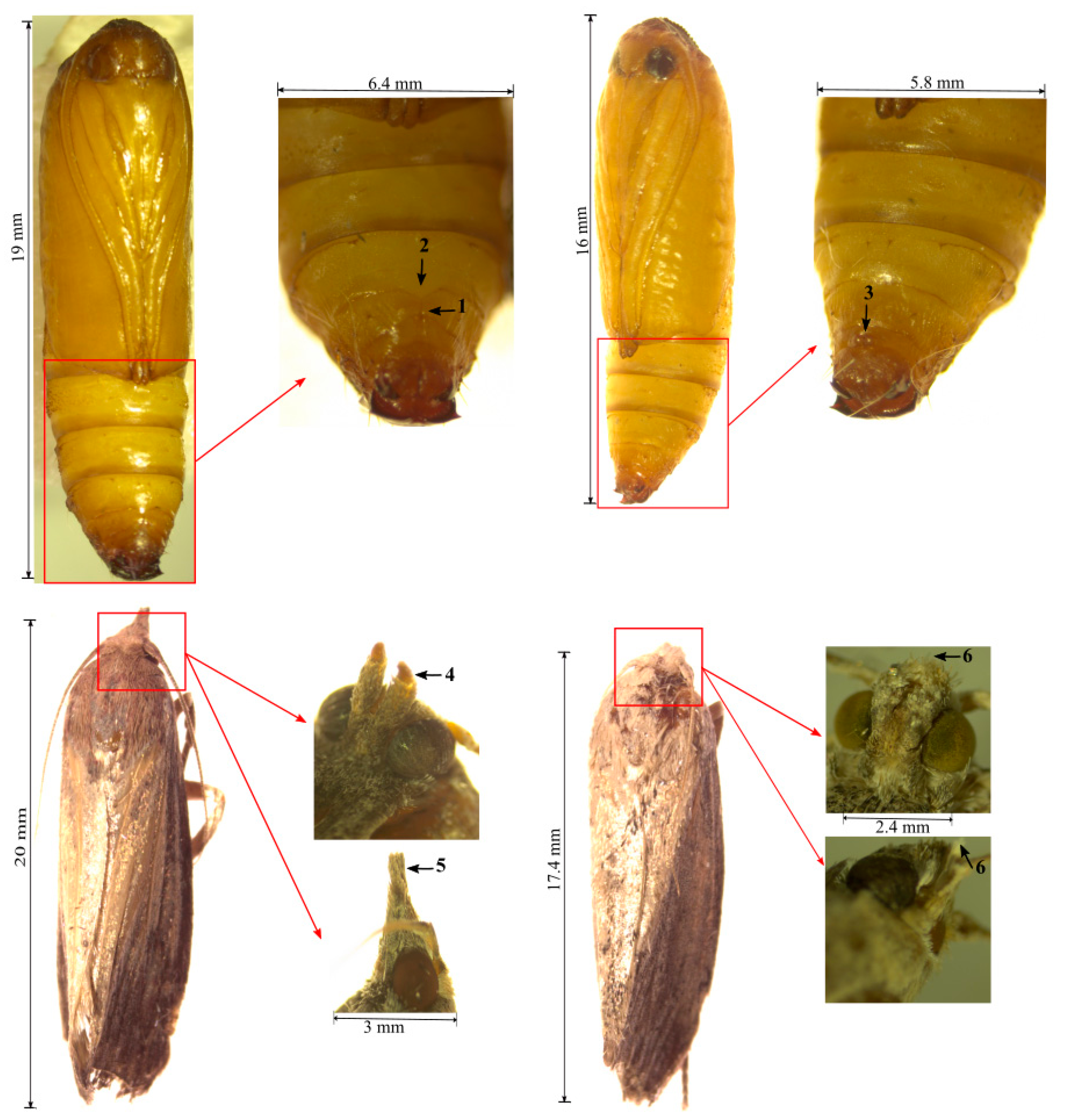The scientific image depicts various developmental stages of a bug, possibly a caterpillar or moth, in a detailed chart format. The image consists of four primary photographs of amber-colored pupae, each accompanied by a close-up of the head and precise measurements. The pupae appear capsule-shaped with distinct lines, indicating an animal's presence inside. Each main image, situated in the corners of the chart, shows the pupa's overall shape and size, while the close-ups highlight specific details like the head. Measurements include sizes such as 19 millimeters long with a 6.4 millimeter head, 16 millimeters by 5.8 millimeters, 20 millimeters with a 3 millimeter head, and 17.4 millimeters with a 2.4 millimeter head. The colors range from yellowish-brown to amber, and the bottom images suggest more mature stages of the pupa, closer to metamorphosis, as they are darker in color. Each section, including isolations of specific parts, combines to form a comprehensive view of the bug's transformation stages.